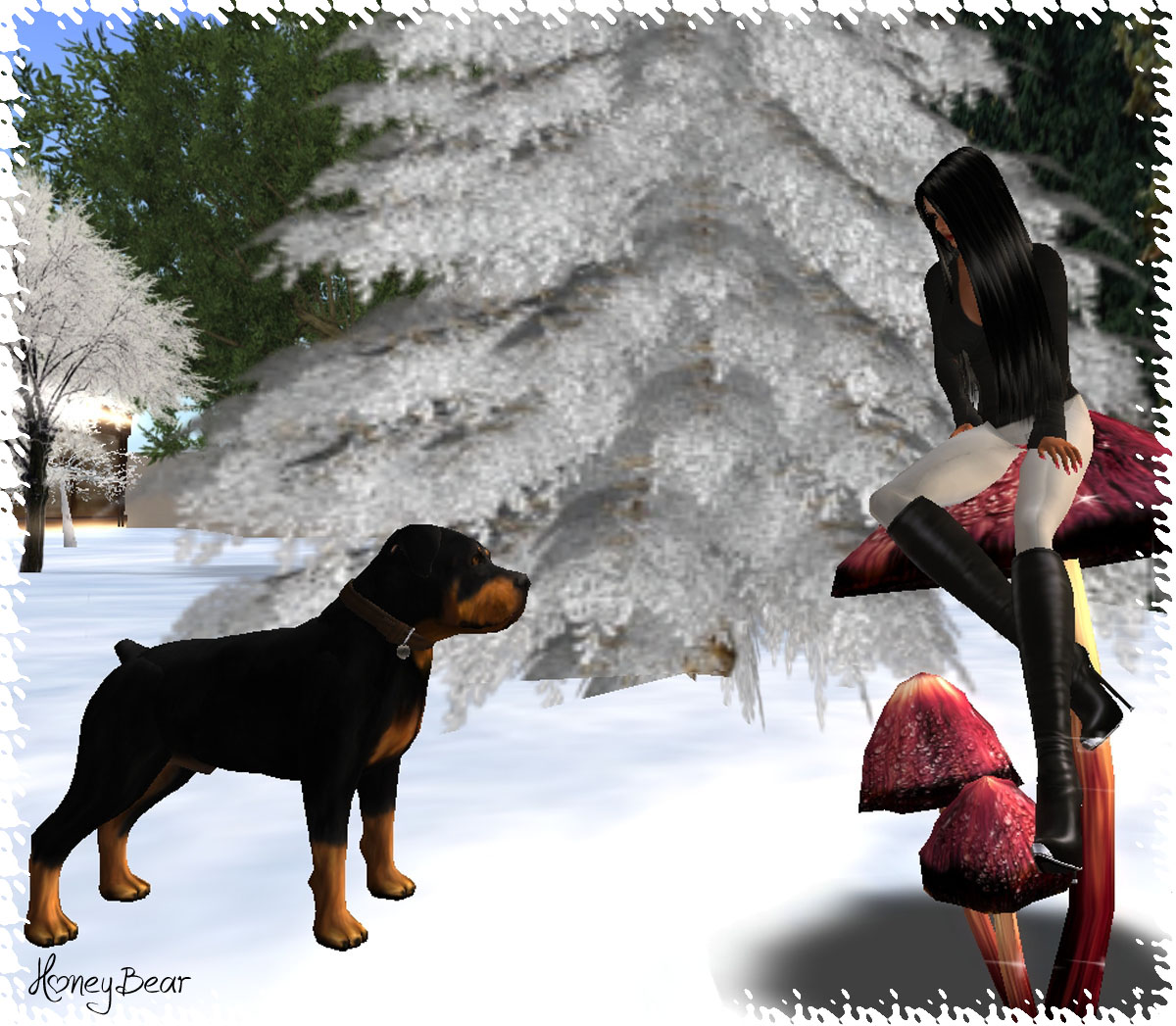In this digitally rendered, winter-themed scene, a woman with long, shiny black hair is seated on a large, maroon-colored mushroom with a yellow and brown base, accompanied by two smaller mushrooms. She is dressed in a black long-sleeved shirt, white leggings, and thigh-high black boots, gazing downward at a Rottweiler-like dog positioned on the left. The dog, predominantly black with brown markings on its face, chest, and legs, is watching the woman intently. The snowy environment features a giant white tree amidst other snow-covered trees in the background, casting a serene, frosty ambiance. The upper left corner showcases a hint of blue sky behind a green, snow-laden pine tree. Additionally, the lower left corner of the image bears the text "Honey Bear," with the "O" stylized as a heart, and the entire image is framed by a delicate, lacy border.